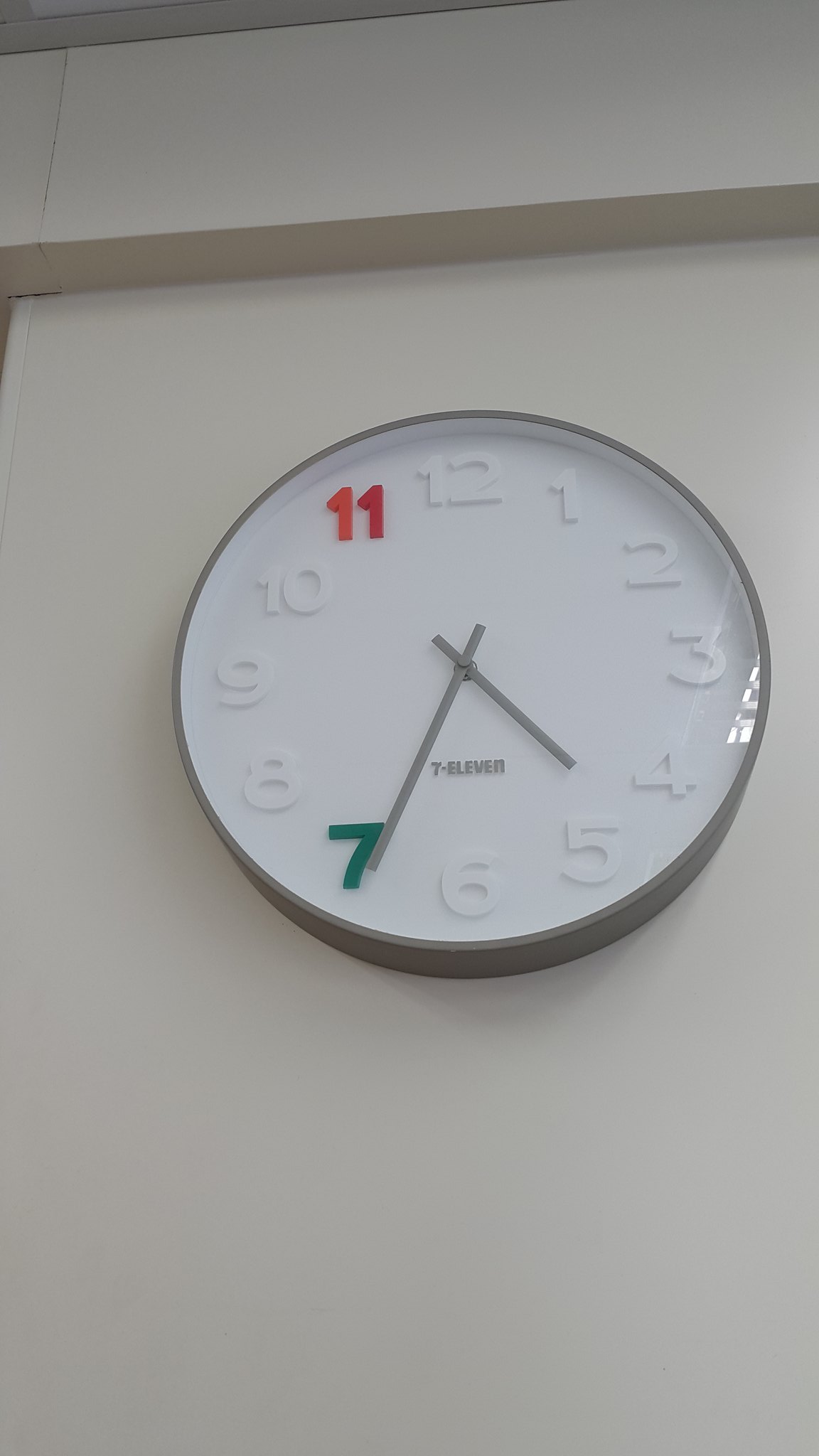This image depicts an analog clock mounted on a plain white wall. Positioned above the clock is a slight ledge that creates an overhang. The clock itself is circular with a white face and is encased in a light gray frame, which could be either plastic or metallic. The numbers on the clock range from 1 to 12, with most being white except for the green 7 at the lower left and the bright red 11 in the upper area. Intriguingly, the 11 is split into two colors—orange on the left side and red on the right. The hands of the clock are light gray, and the text "7-11" is printed in light gray below the center of the clock. Additionally, the clock shows a slight reflection of the ceiling, including some light fixtures, and the time on the clock appears to be around 4:35.